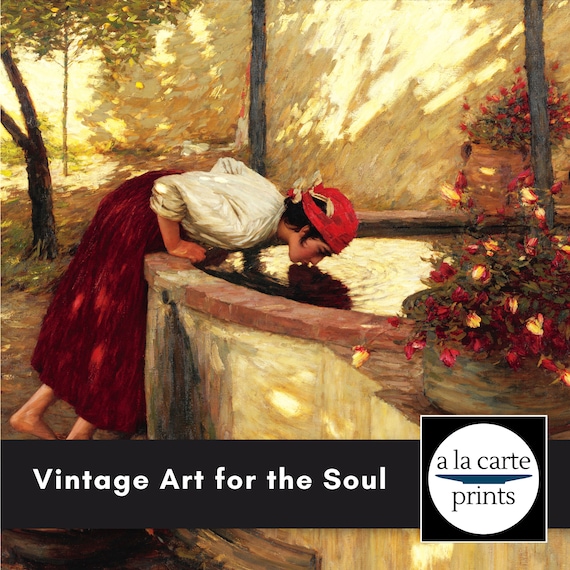The image is a promotional advertisement for an art print shop featuring a watercoloured portrait painting, set outdoors during the daytime, possibly in autumn due to the presence of red leaves on the trees. The scene captures a young woman dressed in a red dress or dark skirt, with a red cap and a white shirt, bending over a waist-high fountain or well, appearing to drink water. The background includes trees and bushes, giving the impression of a serene backyard or garden. To the right of the image, there is a yellow wall, and to the left, an open yard. Roses adorn the right-hand side. At the bottom of the image, white text on a black rectangular background reads "Vintage Art for the Soul," accompanied by a circular white logo with black text that says "Alec Hart's Prints." The artistic representation is slightly blurred, enhancing its vintage feel.